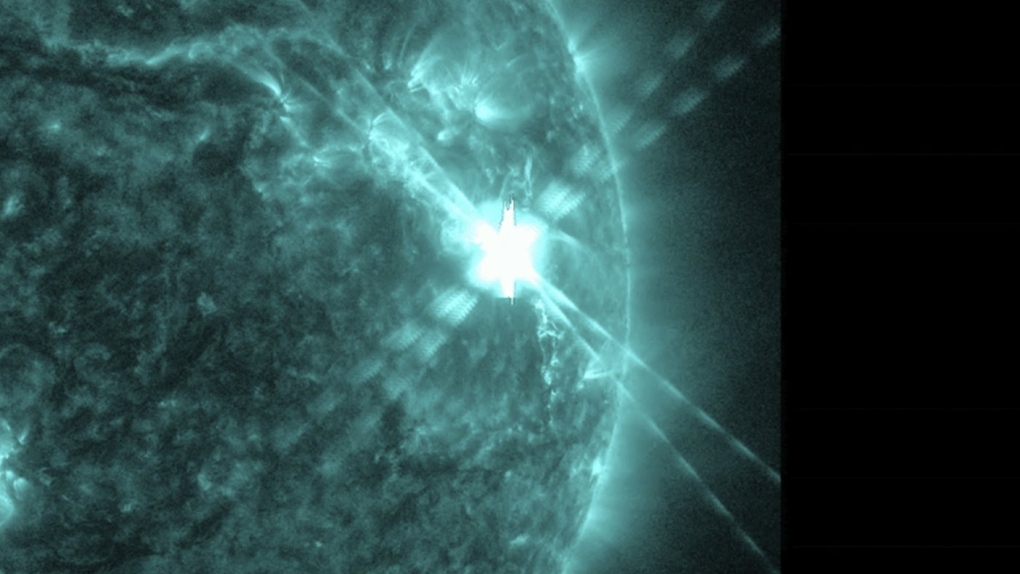The image features a primarily black background with intricate and surreal designs that suggest a science or space-related theme. Dominating the left portion is a partial spherical object that resembles an eye's iris with a bright white center. This spherical shape emits vibrant green and turquoise patterns that radiate outward, somewhat like an x-ray or medical scan, creating an ethereal and futuristic effect. The focal point is a star-shaped object near the center, radiating sharp, bright white lines that intersect to form an X shape. These lines, colored in a gradient blend of light blue and green, shoot off and fade into the surrounding dark background, lending the image a mesmerizing, almost mystical quality. The right side of the image remains predominantly black, providing stark contrast that amplifies the brightness and complexity of the designs on the left. This amalgamation of turquoise, green, and white light patterns against the deep black backdrop makes for a striking and evocative visual experience.